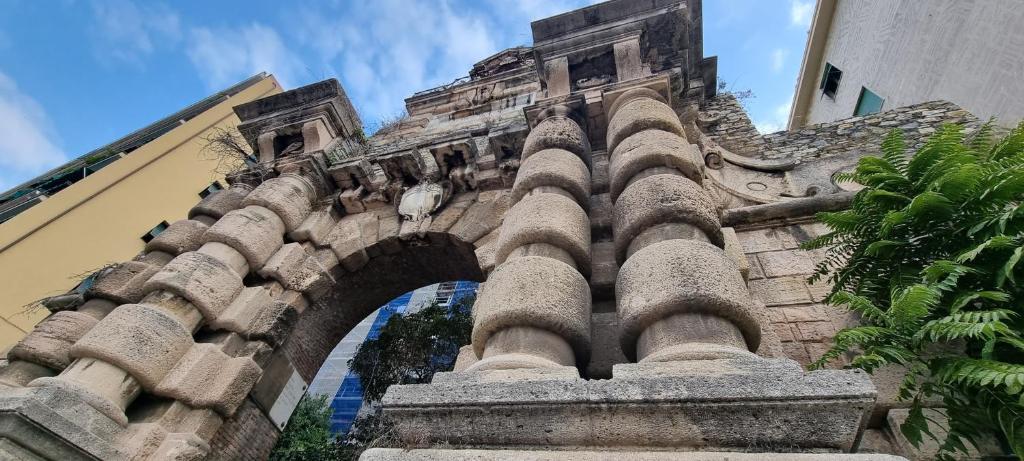The horizontally aligned rectangular image is an upward view from the ground, featuring an older, worn stone structure in the center. The foreground consists of a cement building with numerous vertical columns, each adorned with wristband-like objects. Standing approximately three to four stories high, the main building showcases a large central archway, or cathedral-style opening. Through this archway, a more modern building with windows is visible. Flanking this structure are two other buildings; the one on the left, a taller edifice about six stories high, has a yellowish hue with multiple front-facing windows, while the building on the right is shorter and primarily constructed of grayish-brown stone. The right side of the image also features a touch of nature with green plants or foliage and a tree. Above, the sky is clear blue with scattered, feathery white clouds, completing the vibrant and dynamic composition of the scene.